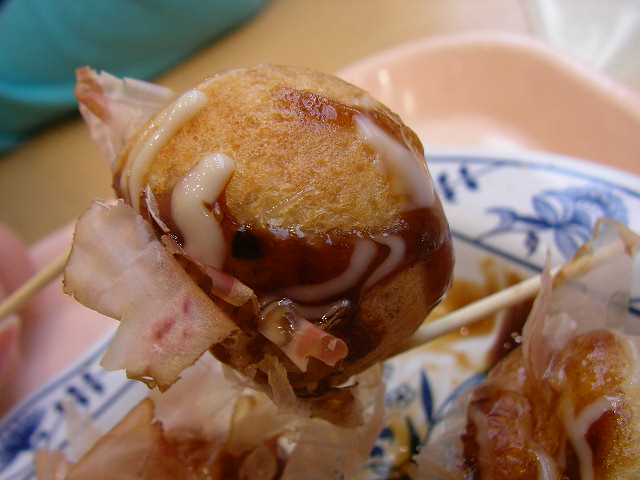The rectangular photograph features a peculiar fried food item being held up, likely with wooden skewers or chopsticks. This enigmatic dish resembles a ball and is drizzled with both a white sauce, which resembles frosting, and a brown sauce that could be barbecue sauce. The surface of the food appears to have some flaky texture, adding to its unusual appearance. 

In the background, a white ceramic plate decorated with blue floral designs is visible, reminiscent of those found in Chinese restaurants. This plate rests on a pinkish-tan plastic tray similar to those used in cafeterias. The close-up shot accentuates the details of the fried ball, leaving its exact nature—whether it's a dessert, a type of savory Asian cuisine, or potentially even wrapped in bacon—ambiguous but intriguing. The overall presentation seems somewhat unappetizing, adding an element of curiosity to the dish.